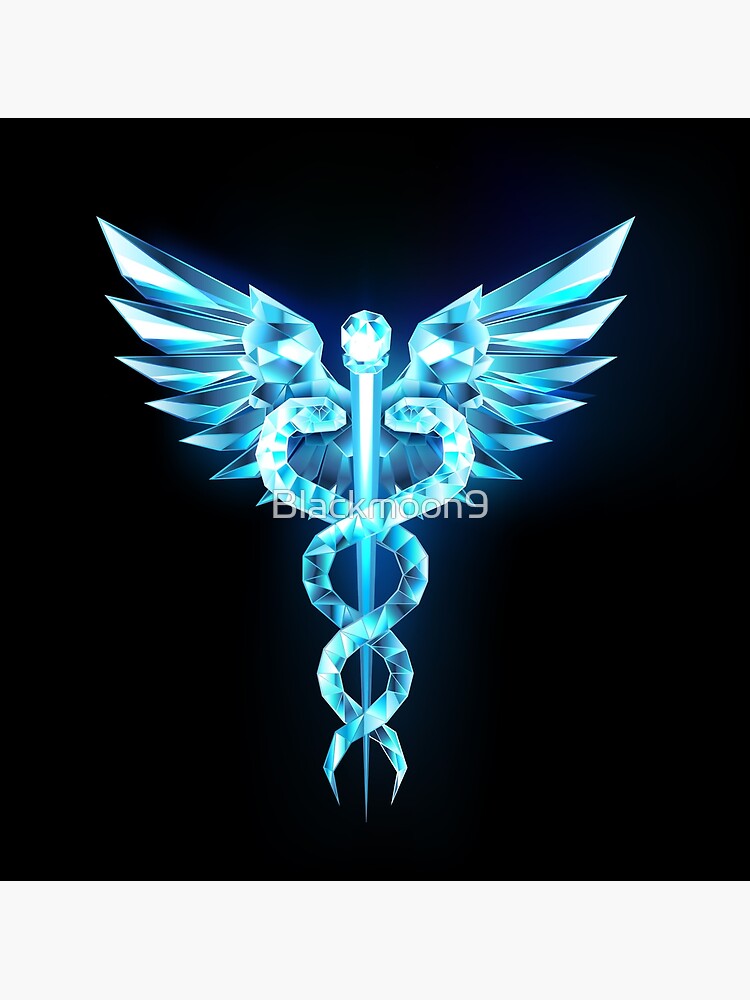The image features a computer-generated, vector-style insignia set against a black background. The centerpiece resembles a medical staff with two serpents intricately wrapped around it, each twisting around the staff twice and facing each other near the top. The staff is adorned with a crystalline, gem-like structure at its apex, with spiky wings extending from both sides just below it. The entire design exudes a blue and white crystal aesthetic. Across the middle of this intricate design, the text "Black Moon 9" is prominently displayed in light gray, with 'B' capitalized and the remaining letters in lowercase, creating a striking and detailed emblem.